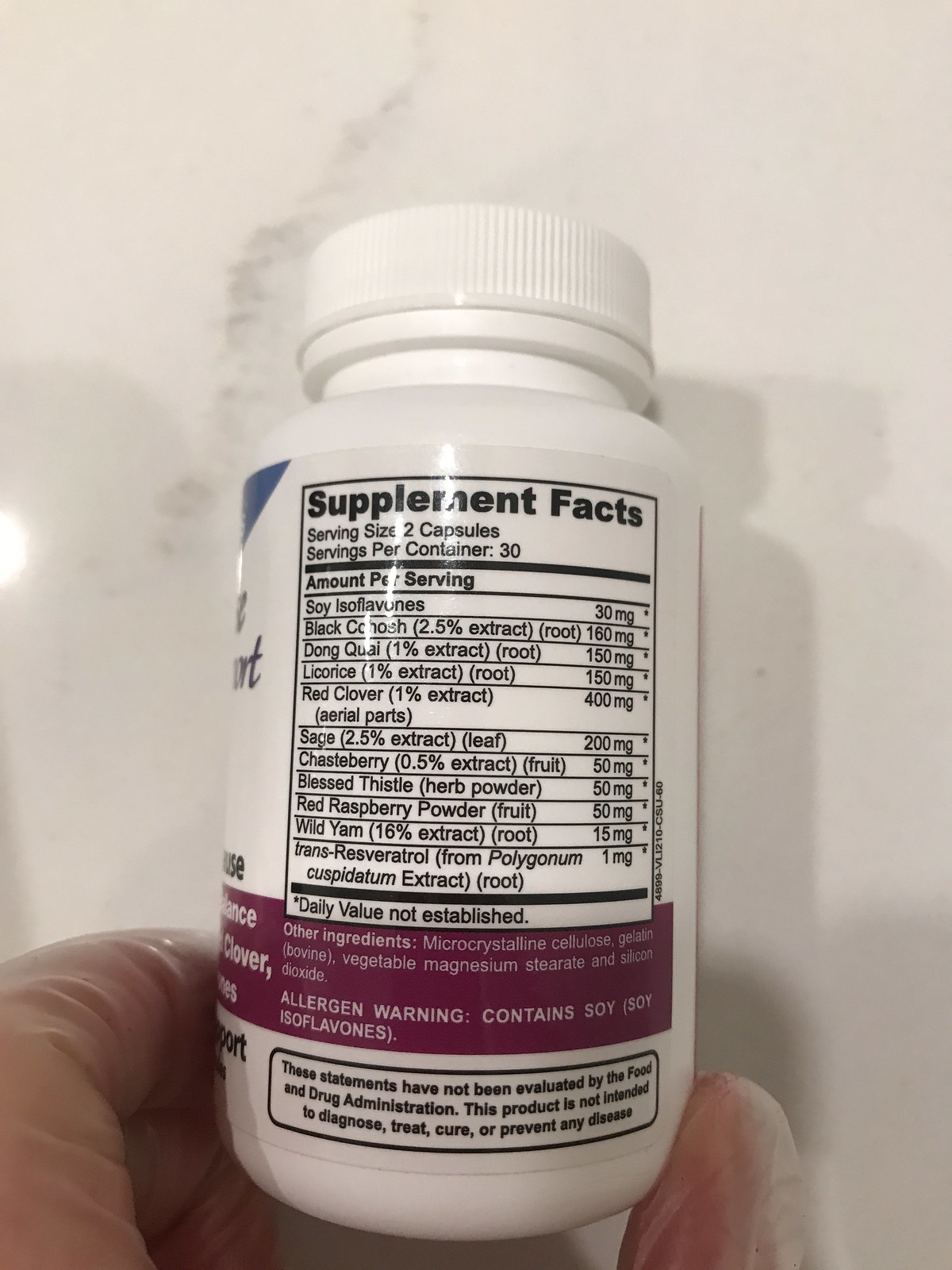A close-up photo captures the back of an opaque white plastic supplement bottle with a white lid, held in the left hand of a person with fair, papery, and wrinkled skin. The bottle is set against a white background, featuring a noticeable gray smudge in the upper left quadrant. The background also appears marble-like with some veining. The bottle’s label, framed by a black rectangular border with purple accents, prominently displays the "Supplement Facts." The serving size is noted as two capsules, with 30 servings per container. Although parts of the text are obscured by glare, the ingredients list includes soy isoflavones, black cohosh root extract, dong quai root extract, licorice, red clover, sage, chasteberry, blessed thistle, red raspberry powder, and wild yam. The allergen warning indicates the presence of soy. Below the facts, a disclaimer states that the product is not intended to diagnose, treat, cure, or prevent any disease. The photograph’s overall composition emphasizes the detailed labeling and the texture of the holder's skin.